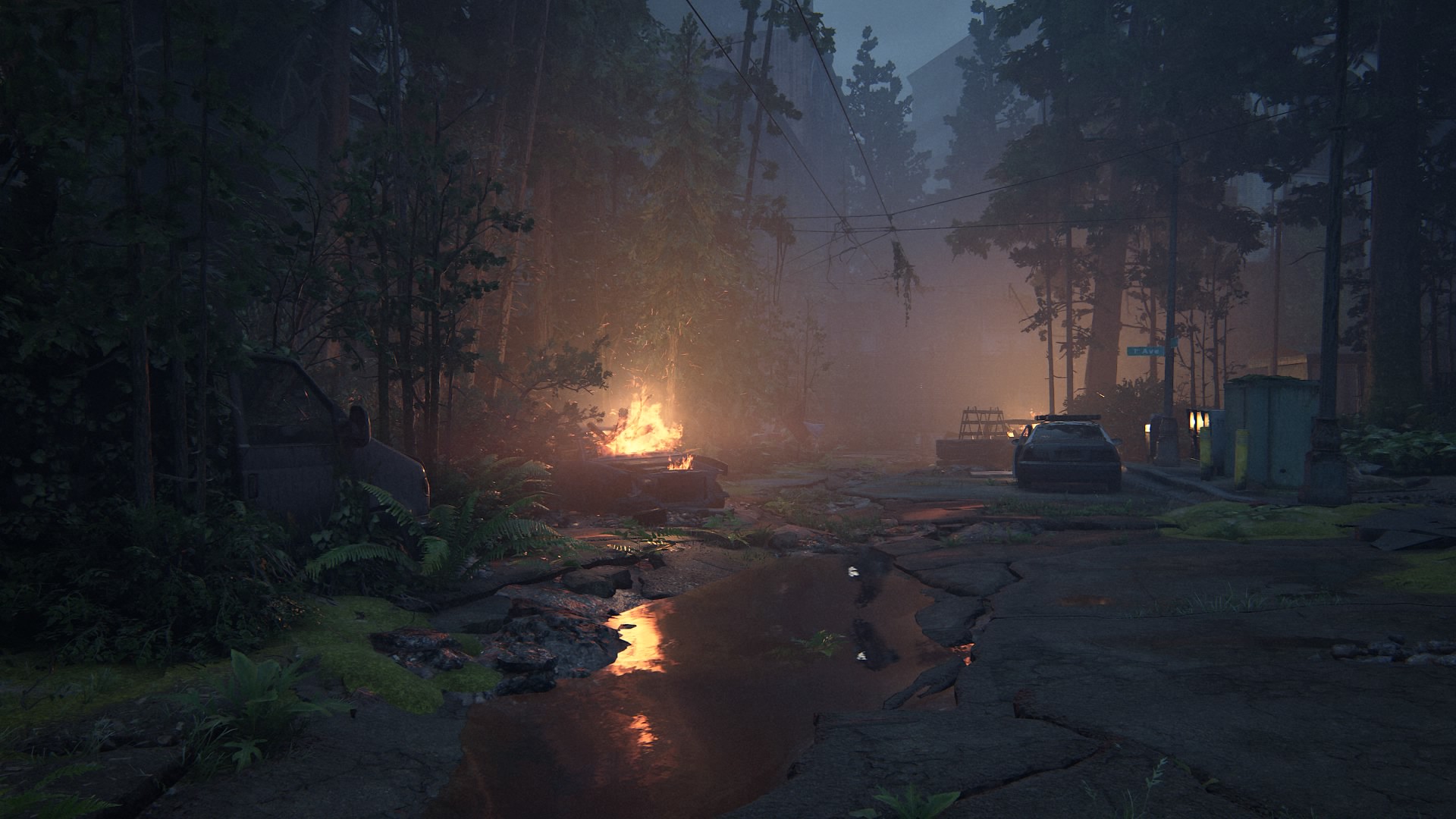In this evocative image, a melancholic, atmospheric scene unfolds within a forested area where nature and remnants of human civilization converge in a milieu reminiscent of a post-apocalyptic setting. At the heart of the composition, a small fire crackles brightly, casting warm light upon the surrounding debris which comprises a rusted car and fragments of a collapsed structure or machinery. The entire scene is shrouded in dense fog or mist, imparting a gloomy and mysterious ambiance. The landscape is rugged and fractured, with moss-covered asphalt fractured and weathered, hinting at prolonged abandonment. Verdant vegetation, including ferns and young trees, has started to reclaim the area, indicating resilience amidst decay. The firelight's vivid reflections shimmer in a puddle on the broken road, adding an element of haunting beauty to this desolate tableau.